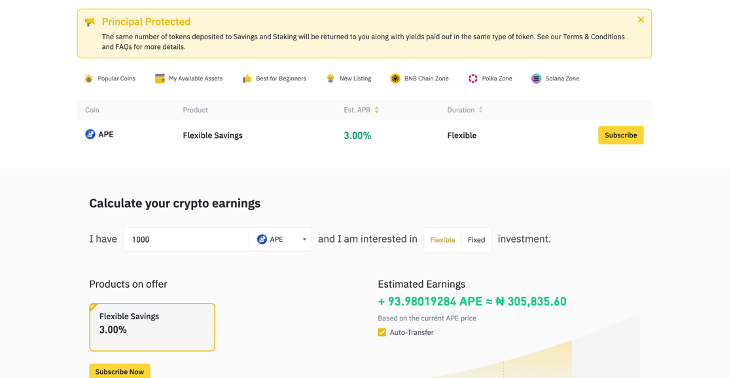In this image, the top section features a primarily pink box outlined in yellow. Within this box, there is a small yellow element on the side accompanied by a hint of blue. The text "Principal Protected" is prominently displayed, followed by a blue line below it.

Beneath this, a set of icons is organized across the top of a blue line, which includes labels such as Coin, Product, Estimated Aim, and Duration. Adjacent to this, there's a small blue circle containing a white arrow.

Below this arrangement, there is the text "APE Flexible Savings 3.00%" followed by the word "Flexible" and a yellow "Subscribe" button. Moving further down, you'll find a blue box titled "Calculate Your Crypto Earnings." 

Within this section, there is an input labeled "I have" displaying "1,000" next to a small blue circle labeled "APE." There are buttons allowing the user to choose between "Flexible" or "Fixed" investments. Below, potential investment products are showcased.

Highlighted is a yellow box with a label "Flexible Savings 3.00%" and another section with an estimated earnings projection plus "93.98019284 APE," totaled out to equal "N305,835.60 based on the current APE price." Finally, a yellow box with a checkmark indicating "Auto Transfer" concludes the detailed description.